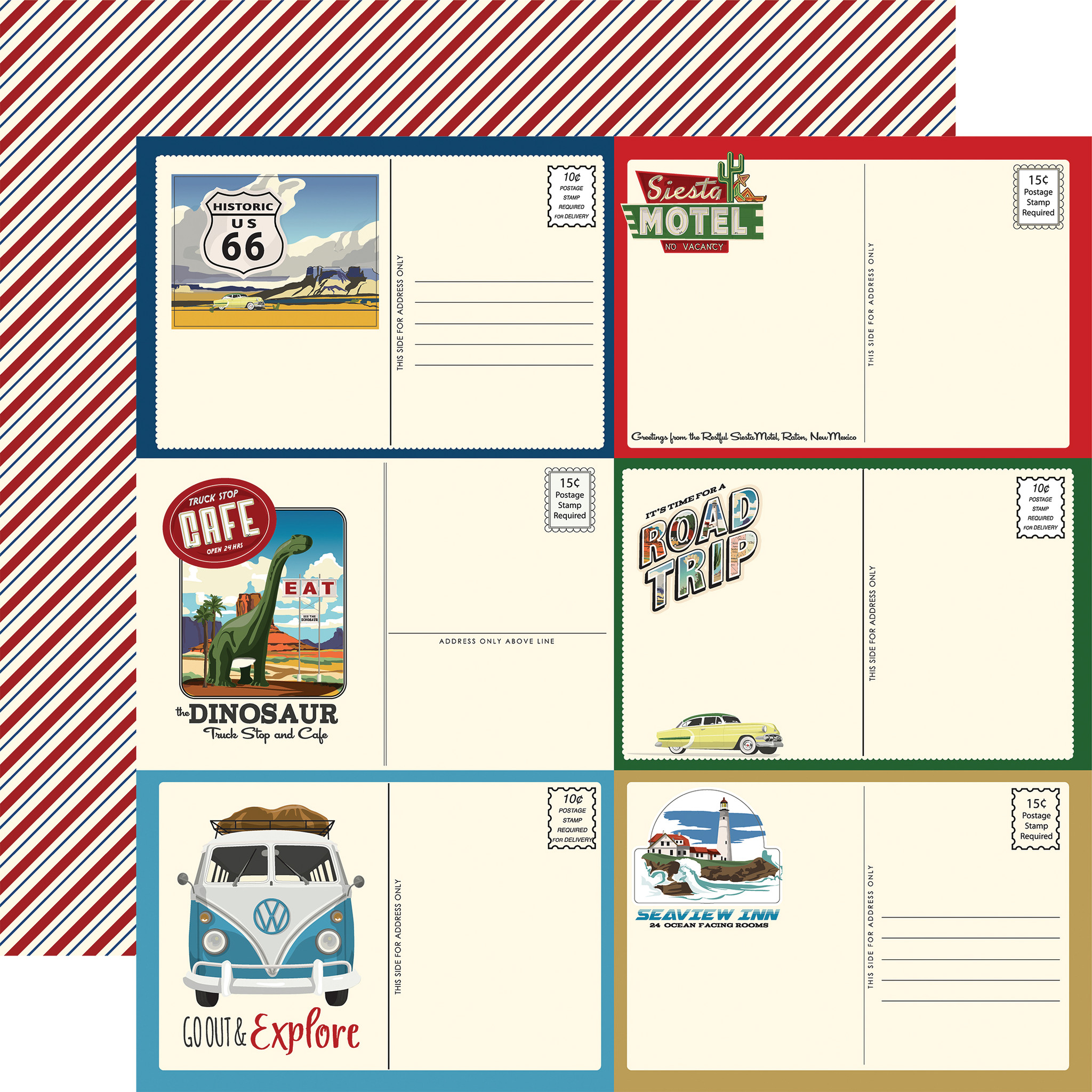This image features a detailed collage of six vintage postcards arranged in two rows and three columns on top of a layered background. The front collage square, approximately 5 inches by 5 inches, showcases various themed postcards, all with a white or beige background and colorful borders in greens, blues, beige, and red. Each postcard is distinct in its design:

1. Top left: "U.S. Historic 66" with a classic car.
2. Top right: "Siesta Motel" with a green cactus.
3. Middle left: "Truck Stop Cafe" featuring a green dinosaur.
4. Middle right: "It's Time for a Road Trip" with a vintage yellow car.
5. Bottom left: "Go Out and Explore" displaying a 1970s Volkswagen van.
6. Bottom right: "Sea View Inn" evoking a lighthouse town similar to those found off the coast of Maine.

Each postcard is designed to mimic the traditional postcard format, with postage values ranging from 10 to 15 cents and spaces for writing addresses and messages.

Behind this collage, there's a second square, slightly offset to the upper left, with a candy cane-striped pattern in alternating diagonal lines of white, red, and blue. This background square enhances the nostalgic and vibrant feel of the image, partially visible around the edges of the postcard collage.